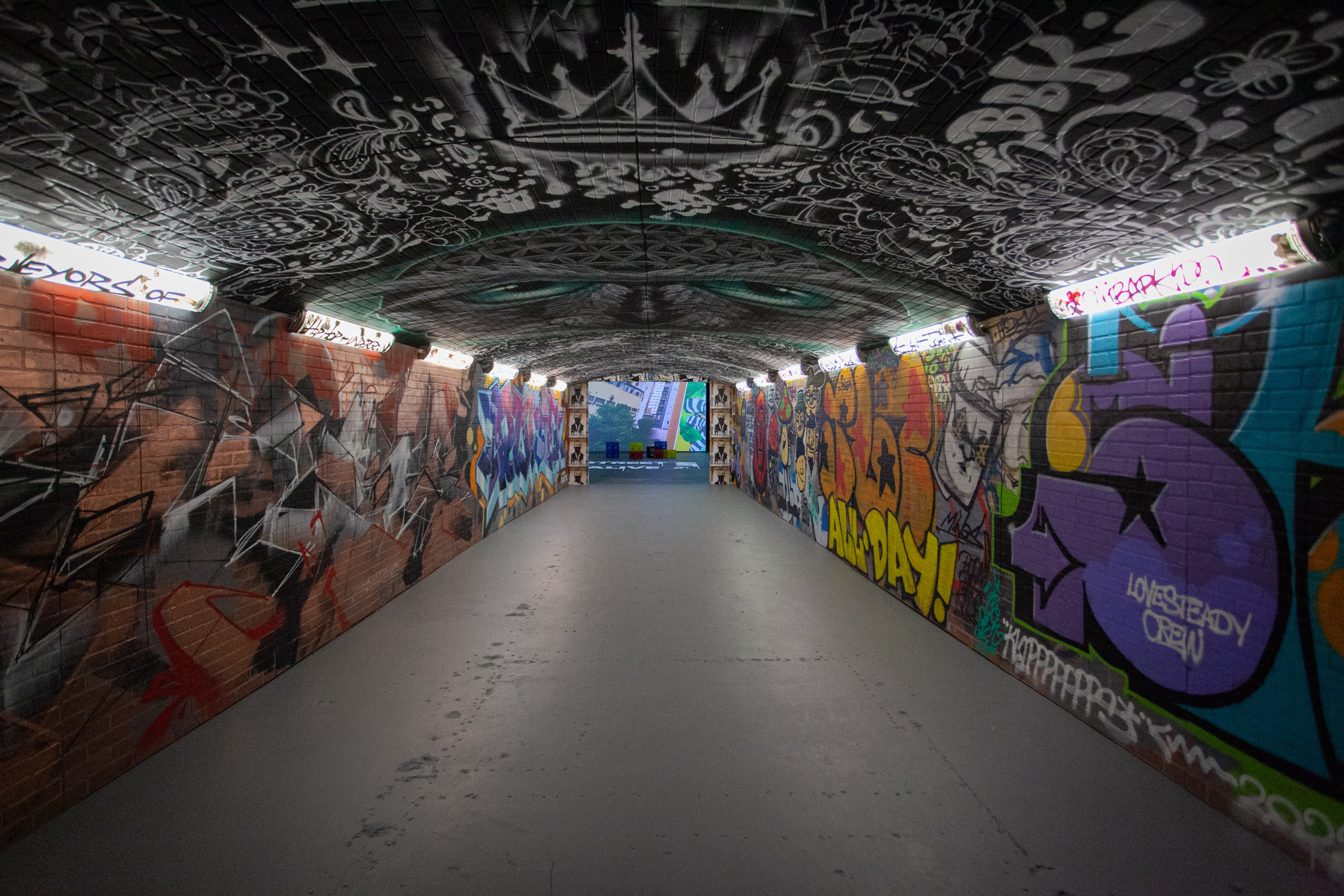This photograph captures the entranceway of an underground tunnel, likely leading to a musical event or bustling lounge in a big city. The tunnel's roof is black and adorned with detailed wall art, including a prominent crown and a mysterious creature with green eyes. Both sides of the tunnel are covered in vibrant graffiti, with the left side predominantly showcasing light red, red, gray, and hints of blue and purple towards the distant end. The right side features a kaleidoscope of colors including purples, yellows, greens, oranges, reds, and blues. Notable graffiti elements include large, hard-to-read letters, with the phrase "all day" visible in yellow towards the bottom. The tunnel is well-lit by fluorescent lights embedded in the ceiling edges, ensuring that the vivid artwork is easily viewable and the concrete pathway is safely navigable.